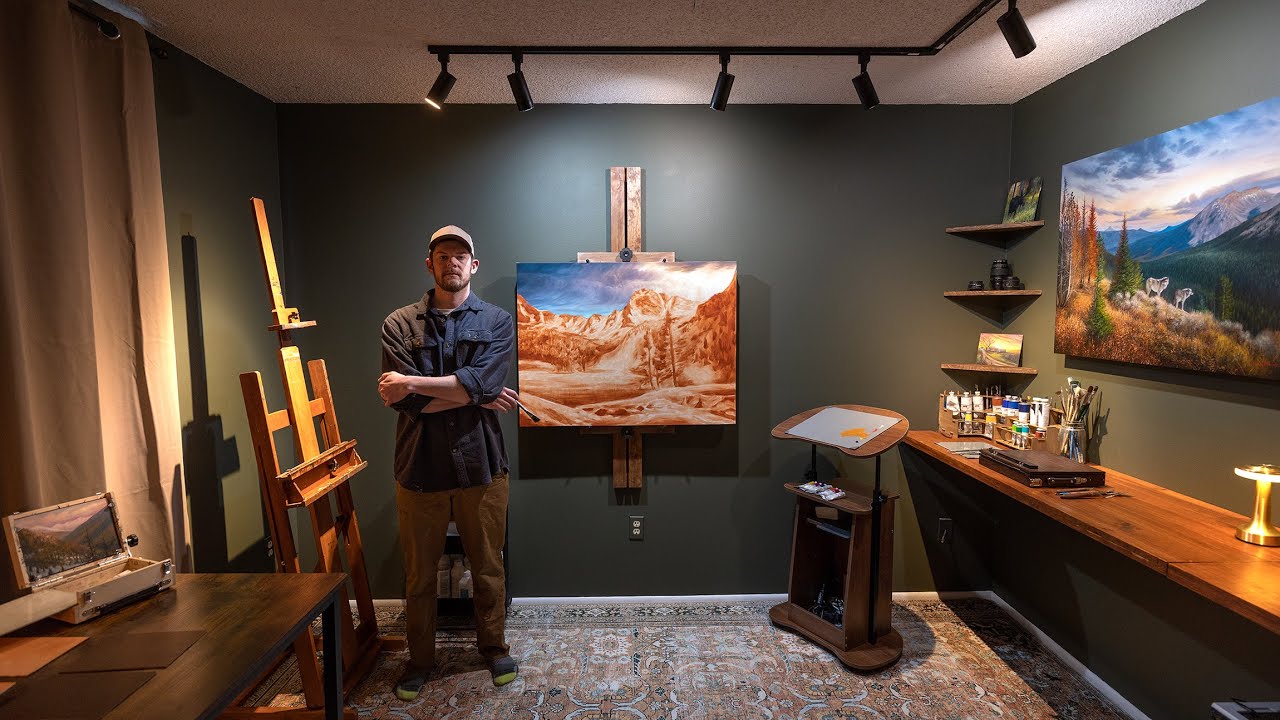In this detailed color photograph, an artist stands confidently in his studio, arms crossed and facing the viewer. He wears a white baseball cap, a dark blue button-down shirt, and tan pants, completed by socks with colored tips, standing on an oriental-style rug. The studio walls are painted a deep charcoal color, contrasting with a white ceiling equipped with black track lighting, featuring five to six adjustable downlights.

To the artist's left, there's an empty wooden easel casting a shadow against the wall, matched by an open wooden table holding a box. Adjacent to this setup is a long white curtain that flows to the floor. Above the artist, numerous art supplies, including paints and brushes, populate a shelf, ensuring that all necessary materials are within easy reach.

Directly to the artist's right stands a large easel displaying a vibrant desert landscape painting. The artwork captures a canyon under a blue sky dotted with clouds, featuring sandy terrain flanked by rugged hills. Below this painting, an electrical outlet is barely visible.

Further right, a long table supports bottles of paint, brushes, and other miscellaneous artistic tools. Another eye-catching painting mounted on the wall depicts two wolves standing on a hill overlooking a valley and mountaintop. In the corner, a three-tiered shelf houses a variety of items, including a painting of a moose, a small golden lamp, and a closed briefcase, with smaller shelves displaying indecipherable objects and another landscape painting.

The overall scene captures the essence of a dedicated artist deeply embedded in his creative environment, surrounded by tools of his craft and inspiring works of art.